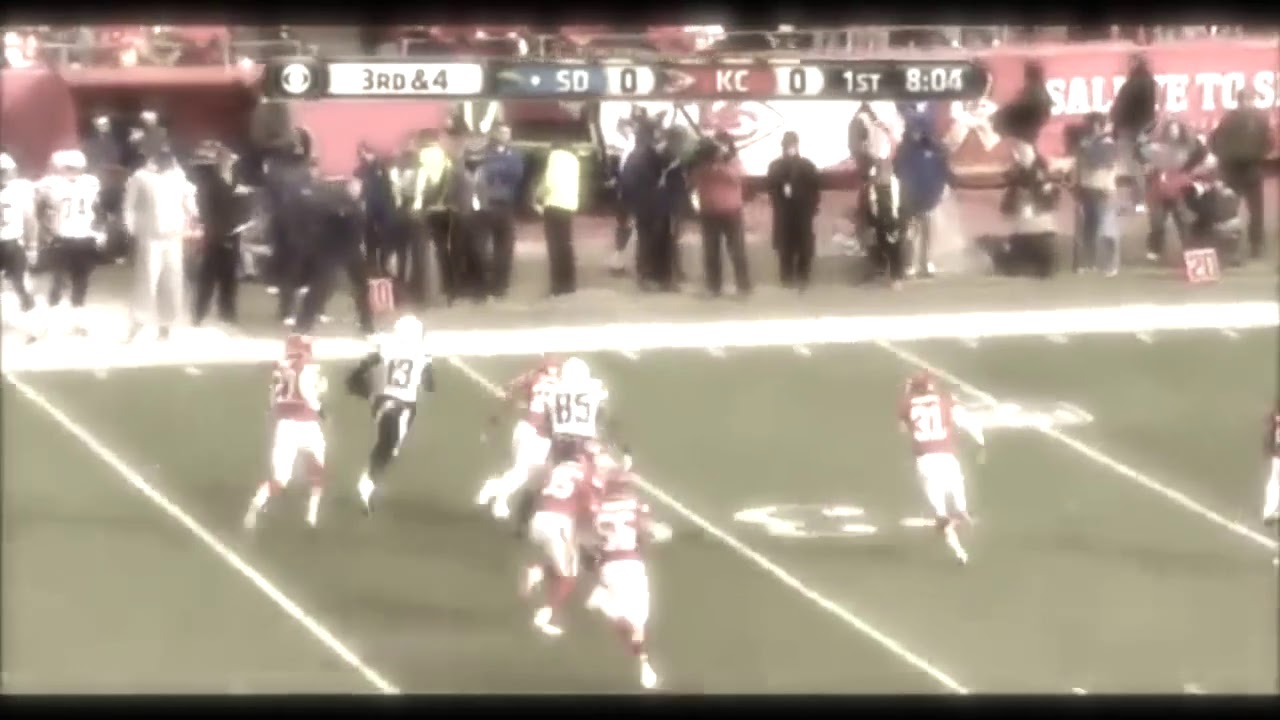This is a brightly filtered screenshot from a video of an American football game featuring the Kansas City Chiefs (KC) and an unspecified team in dark green (SD). The image, captured from an elevated angle approximately 10 feet above the field, showcases players in red and white jerseys in mid-motion, running towards the right side of the field. Visible players are numbered 27, 13, 85, 56, and 31. Surrounding the field are standing individuals, including spectators, camera crews, coaches, and other players waiting for their turn. The top section of the image displays a scoreboard with the text: "3rd and 4th, SD 0, KC 0, 1st & 8:04". Additional visual details include green grass with customary field lines and banners along the sidelines featuring logos and brand names.